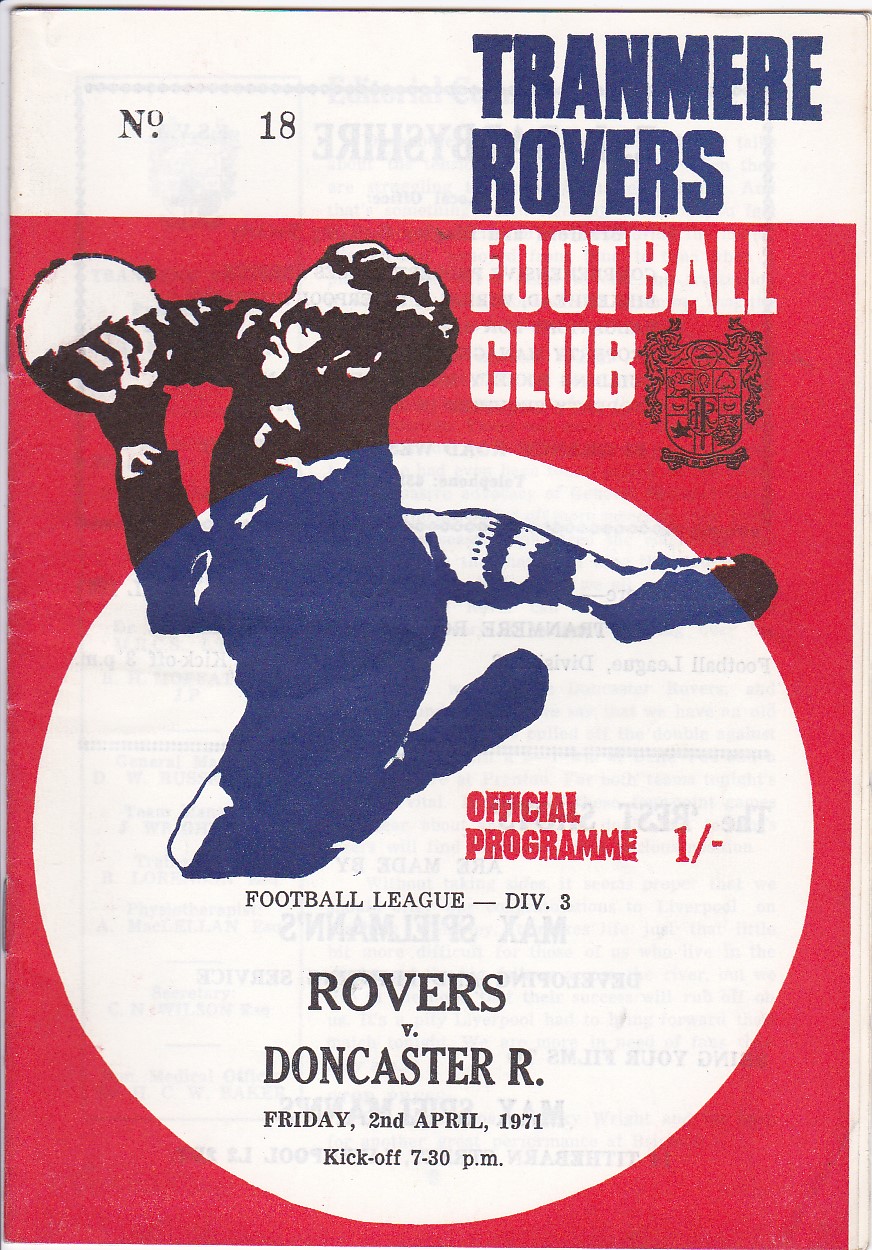This is the front cover of an official program for a soccer event featuring the Tranmere Rovers Football Club. Positioned centrally, the cover showcases a large red rectangle background with a white circle in the center. Inside the circle, there is a detailed drawing of a soccer player, likely a goalie, depicted in action as he jumps to catch the ball. Above the illustration, the text prominently reads "No. 18, Tranmere Rovers Football Club," in a mix of white and blue fonts. Below the image, in black and white text, it states "Official Program 1 - Football League Division 3," followed by "Rovers v. Doncaster R," all in capital letters. The date and time of the event are specified as "Friday, 2nd April 1971, kickoff 7.30 p.m." The overall design is visually engaging, utilizing a color scheme of blue, red, and white, with the illustration adding a dynamic element to the program cover.